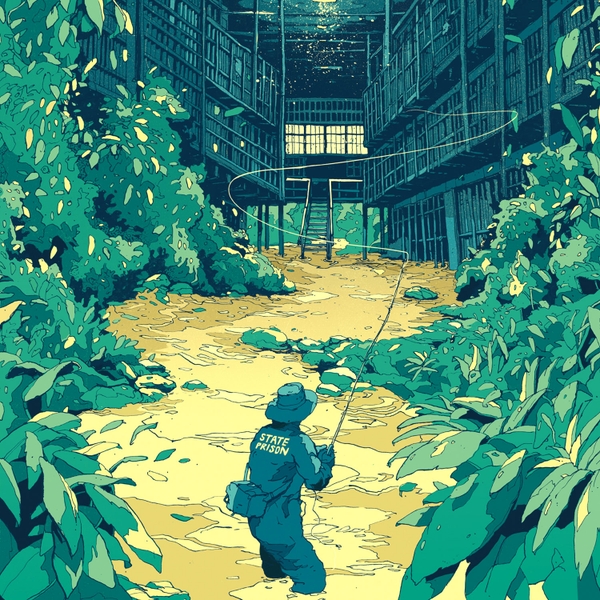The image is a detailed piece of digital art or a drawing depicting a surreal prison scene. At its center is a man standing knee-deep in a yellow liquid, wearing a long-sleeved one-piece outfit that reads "state prison" in yellow text on his left shoulder and back hip. On his back hip, he carries a box-like tackle box, adding to his fisherman's appearance, which is further emphasized by the round fisherman's hat on his head. In both hands, he holds a fishing rod, with the fishing line extending upwards toward various prison cells in a multi-level block. The floor of the prison cells is submerged in the same yellow liquid in which the man stands. Surrounding the scene on either side are tall green bushes, with leaves falling off, creating a sense of decay. In the background, a staircase can be faintly seen, adding depth to the prison setting. The colors in the artwork range from dark greens and regular greens to yellows, grays, and blacks, creating a somber, surreal atmosphere.